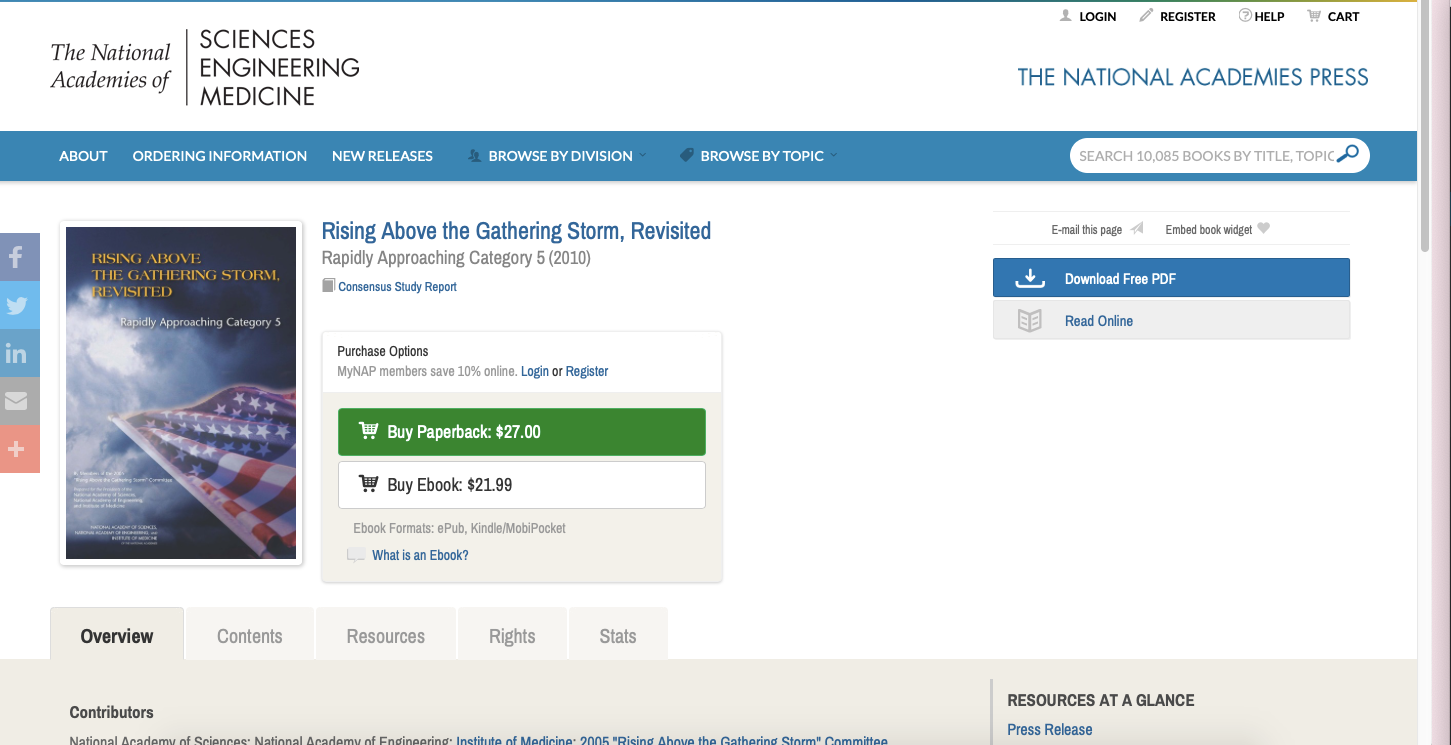The image depicts the homepage of the National Academies Press website. At the top of the page, the banner displays the titles "National Academies of Sciences, Engineering, and Medicine," along with the National Academies Press logo on the right. The top navigation bar includes options to log in, register, access help, and view the shopping cart.

Below the main banner, a blue navigation bar stretches across the width of the page, featuring clickable options: "About," "Ordering Information," "New Releases," "Browse by Division," and "Browse by Topic." At the end of this row, a white search bar with the placeholder text "Search 10,000 books by title topic" is visible.

The main section of the page showcases a featured book titled "Rising Above the Gathering Storm, Revisited," categorized under "Category 5 of 2010." The book is available in paperback for $27 and as an e-book for $21.99. On the left-hand side, a vertical column of social media icons allows users to share content across various platforms.